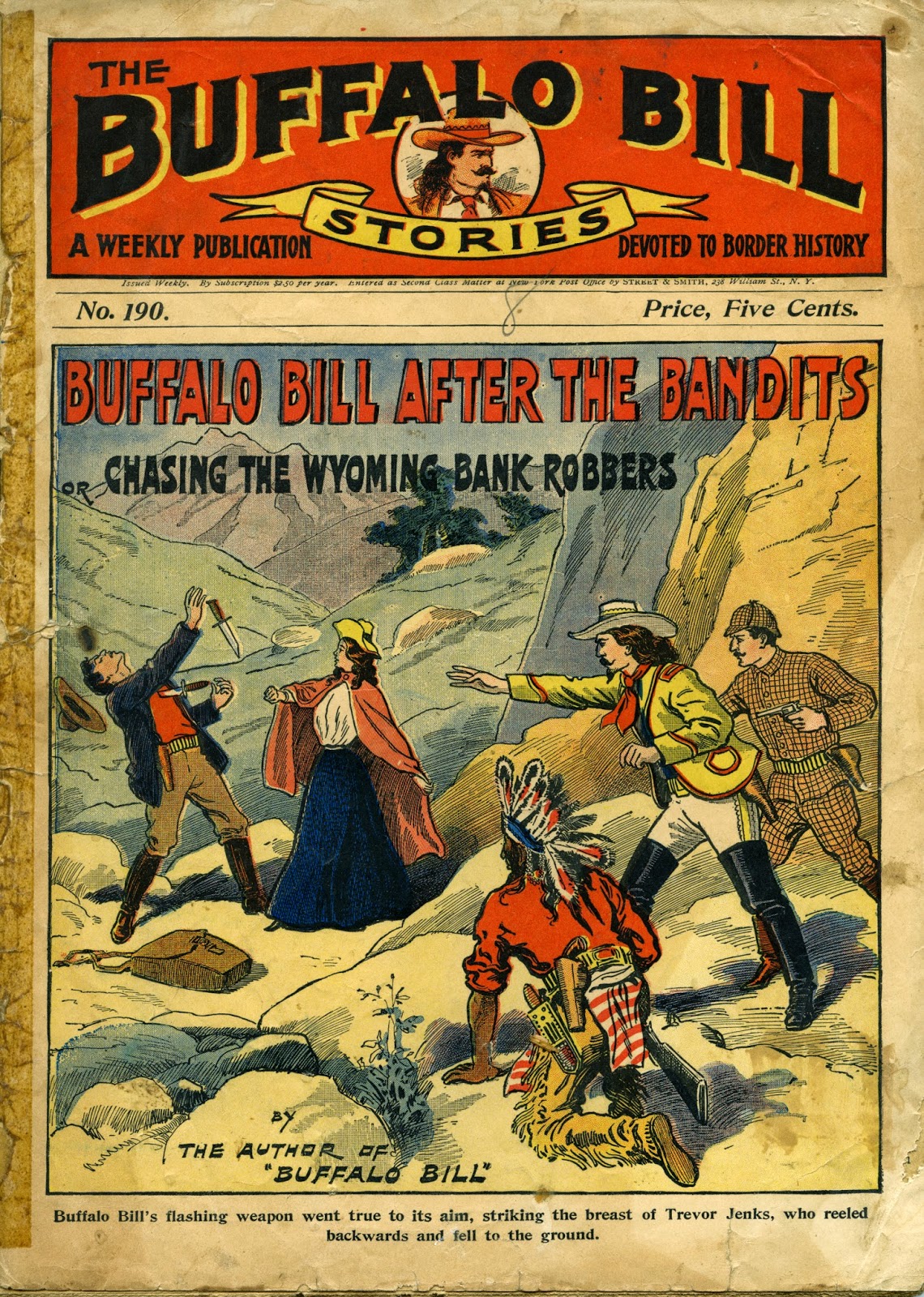The cover of a comic book titled "The Buffalo Bill Stories" features a pale yellowish-brown background and has a logo at the top with a red background and black text, partially highlighted with a yellow drop shadow. The top reads, "The Buffalo Bill Stories: A Weekly Publication Devoted to Border History," with the issue number 190 and the price of 5 cents spelled out on the right side. Central to the cover, an oval portrait of a man, presumably Buffalo Bill, with long dark hair, an orange hat, and an orange necktie stands out. The main title, "Buffalo Bill After the Bandits, Chasing the Wyoming Bank Robbers," is prominently displayed in bold red text, with surrounding captions in black. The illustration below depicts an intense scene: Buffalo Bill lashes his weapon, striking a man identified as Trevor Jenks in the chest, causing him to reel backward and fall. To the forefront, a Native American warrior, wearing red with feathers in his cap, kneels, while to the right side, Buffalo Bill, a native figure, and another man in a brown uniform with a gun, observe the unfolding drama.